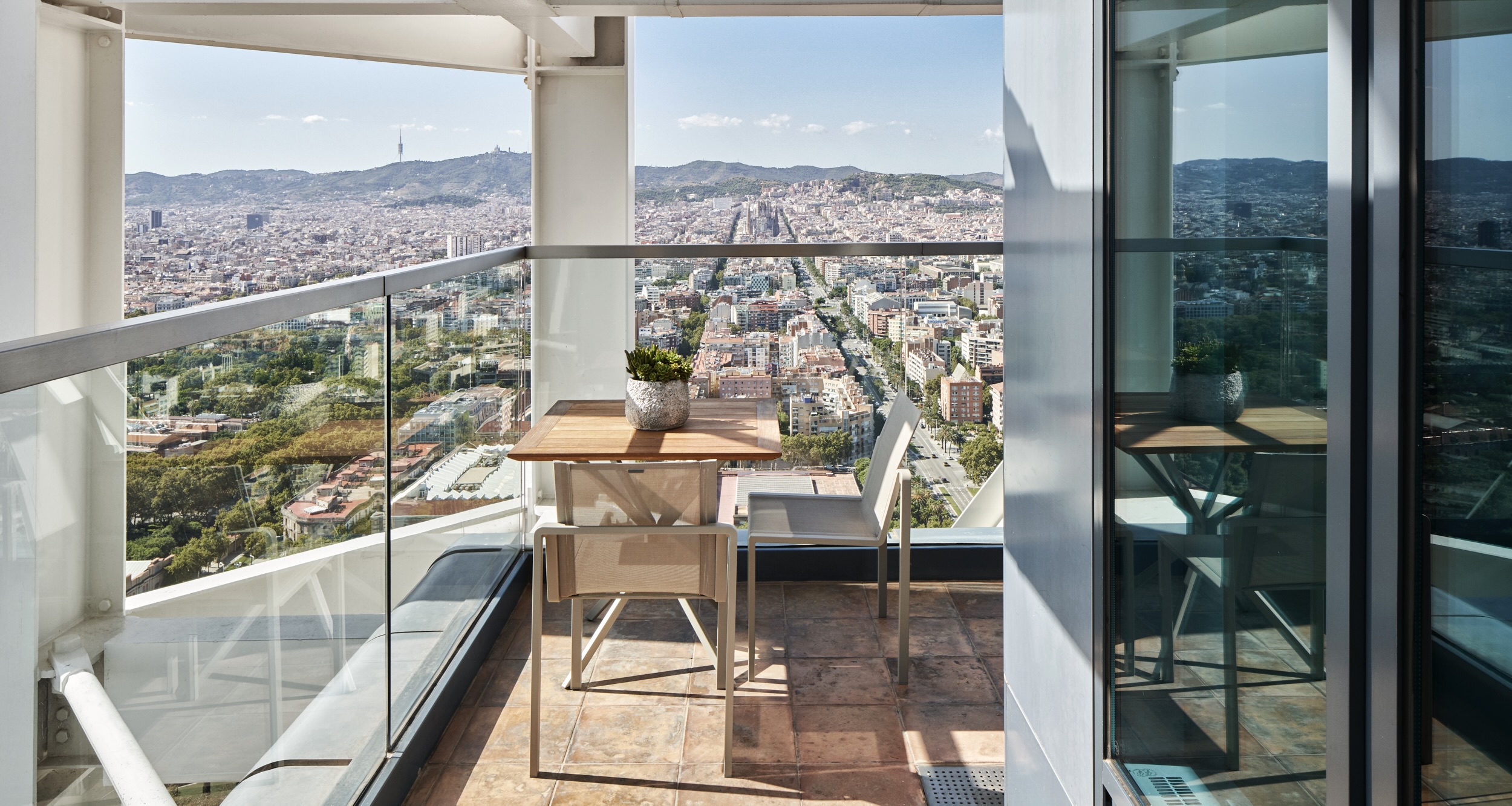The photo depicts a vibrant cityscape viewed from an elevated and refined apartment patio. The high vantage point, possibly not the very top floor but still significantly high, offers an expansive view of the bustling city center with rooftops stretching to the horizon and a clear, bright blue sky overhead. Distant mountains and patches of greenery, including a park to the side, complement the urban scene. 

The modern patio features glass panels with metal framing instead of conventional railings, providing an unobstructed view. A simple wooden table is positioned centrally with minimalist white metal and fabric chairs surrounding it. Atop the table sits a solitary plant, enhancing the tranquil outdoor space. The patio connects to the apartment's interior through sleek glass sliding doors, which reflect the outdoor furniture.

The apartment's structure has noticeable industrial elements, with visible metal beams adding to its contemporary aesthetic. The atmosphere is bright and sunny, with sunlight highlighting the greenery to the left and illuminating the reflective surfaces and white walls within the space. This combination of elements creates a serene yet dynamic urban retreat.